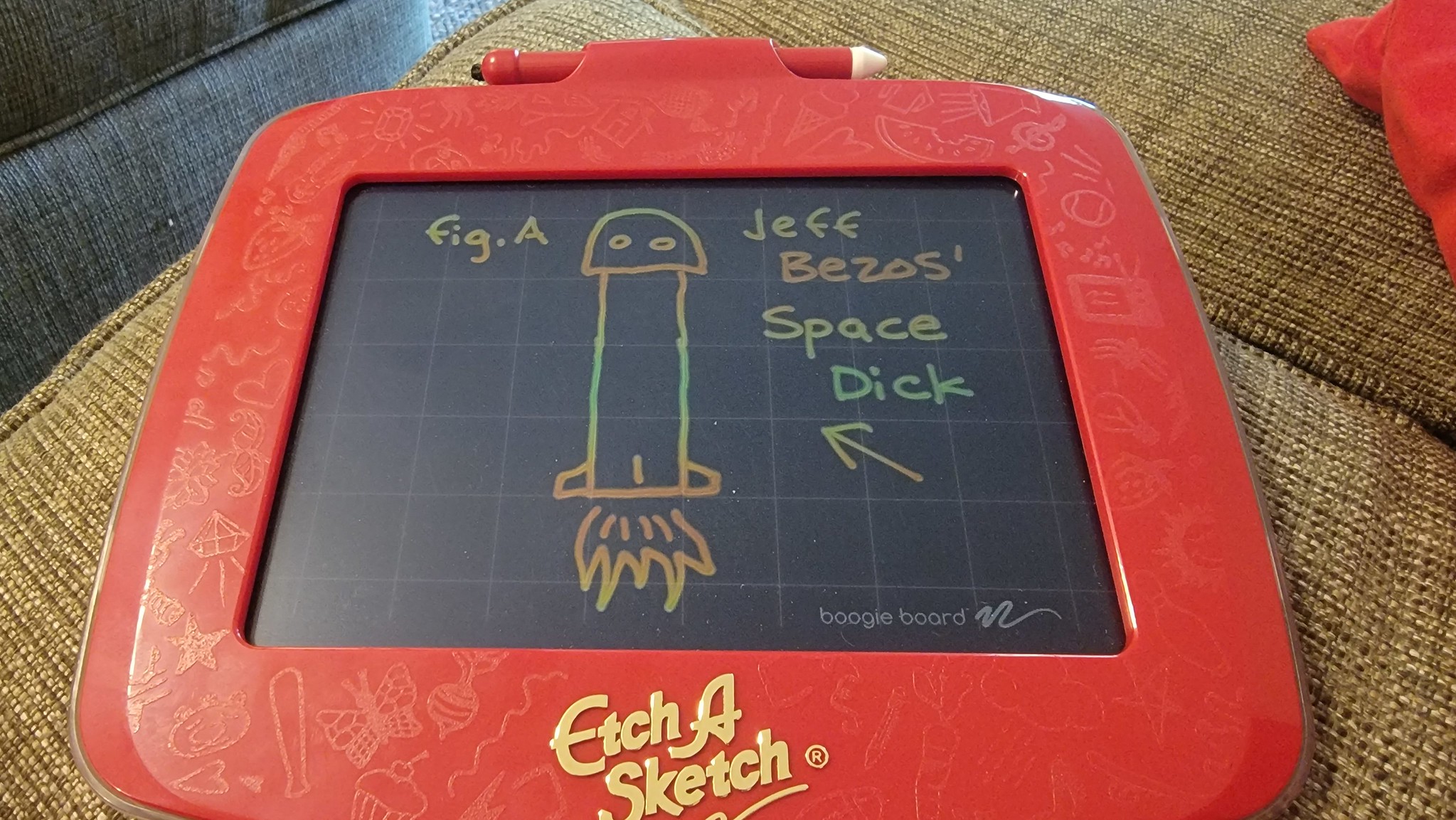This humorous piece on a rainbow Etch-a-Sketch depicts a caricature of Jeff Bezos' rocket, styled in a manner reminiscent of male anatomy. The artwork emphasizes the phallic appearance of the spacecraft famously launched by Bezos. In a playful and lighthearted manner, it captures the absurdity and humor often associated with the rocket's design. The etching is detailed, showing great effort in mocking the eccentricities of modern space exploration. Additionally, some text—possibly incomprehensible or stylized as "fig-a" or "e-i-g dot-a"—accompanies the drawing, adding a quirky touch to the overall image. This creative satire is an unexpected but amusing commentary on contemporary space travel, reflecting a clever sense of humor.